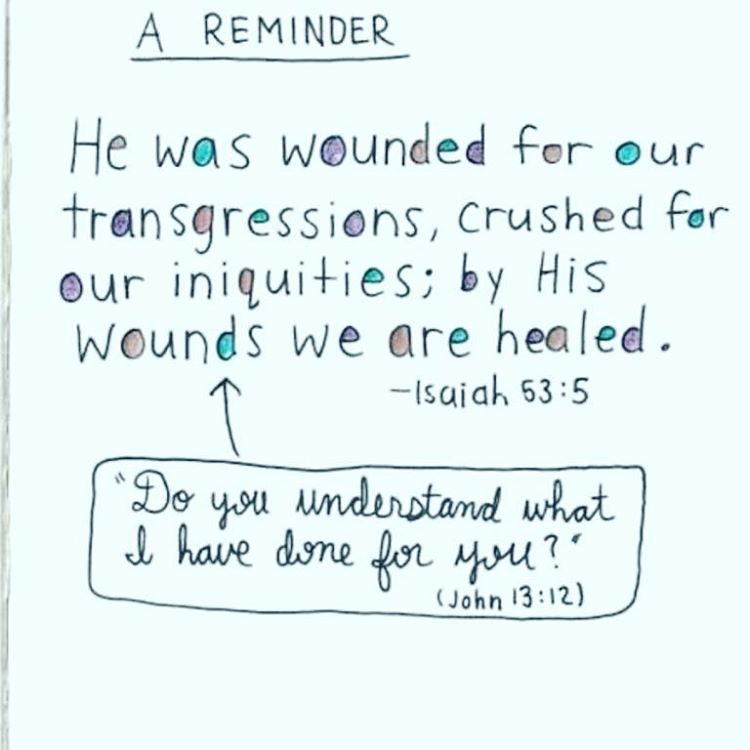The image depicts a seemingly photocopied blue sheet of paper with a handwritten message prominently displayed in the center. The background appears slightly blurry and white, adding to the simplicity of the setting. The text, written in blue and varying other shades, reads as follows:

At the top, in caps and underlined, it says, "A REMINDER." Below this header, the main body of text reads, "He was wounded for our transgressions, crushed for our inequities; by His wounds we are healed." This is followed by a dash and the reference "Isaiah 53:5" on the right side. Further down, enclosed by a hand-drawn box with an arrow pointing to the word "wounds," another line states, "Do you understand what I have done for you?" with the citation "John 13:12" in parentheses beneath it. Notably, some of the letters, like the 'A' and 'O,' are filled in with colors such as teal and purple, adding a subtle yet intriguing detail to the otherwise monochromatic blue text.

The overall aesthetic of the image suggests it might be a reflective or devotional piece, likely to be found inside a church or a place meant for contemplation.